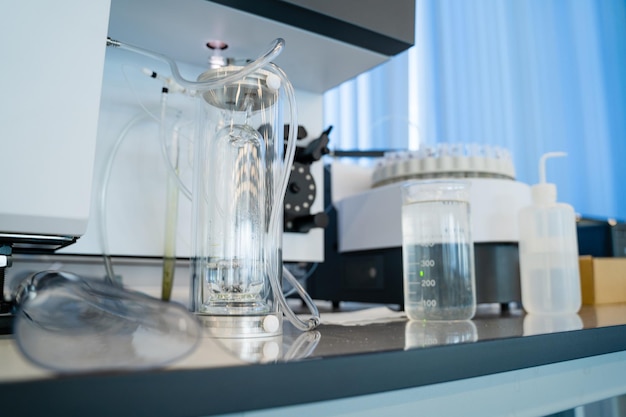In this detailed image of a chemistry or scientific laboratory, we can see a variety of laboratory equipment arranged on a black, science-classroom-like counter, captured from a downward angle. Dominating the scene slightly left of center is a thick, clear glass bottle with a stopper at its top, perforated to allow flexible tubes to pass through, connecting it to an adjacent piece of machinery. To the right of this glass bottle, there is a clear container with measurement markings, filled with liquid, accompanied by a small plastic squirt bottle with a spout. 

The table also features a centrifuge, identifiable by its black and white plastic construction, possibly holding test tubes and situated under a larger rectangular chemical apparatus, of which only part is visible. A pair of safety goggles is partially obscured in the bottom corner of the frame. Above the laboratory setup is a cabinet with a dark gray front and a white underside. The background reveals a blue curtain, adding a subtle artistic touch to the picture, which provides an additional layer of depth and context.